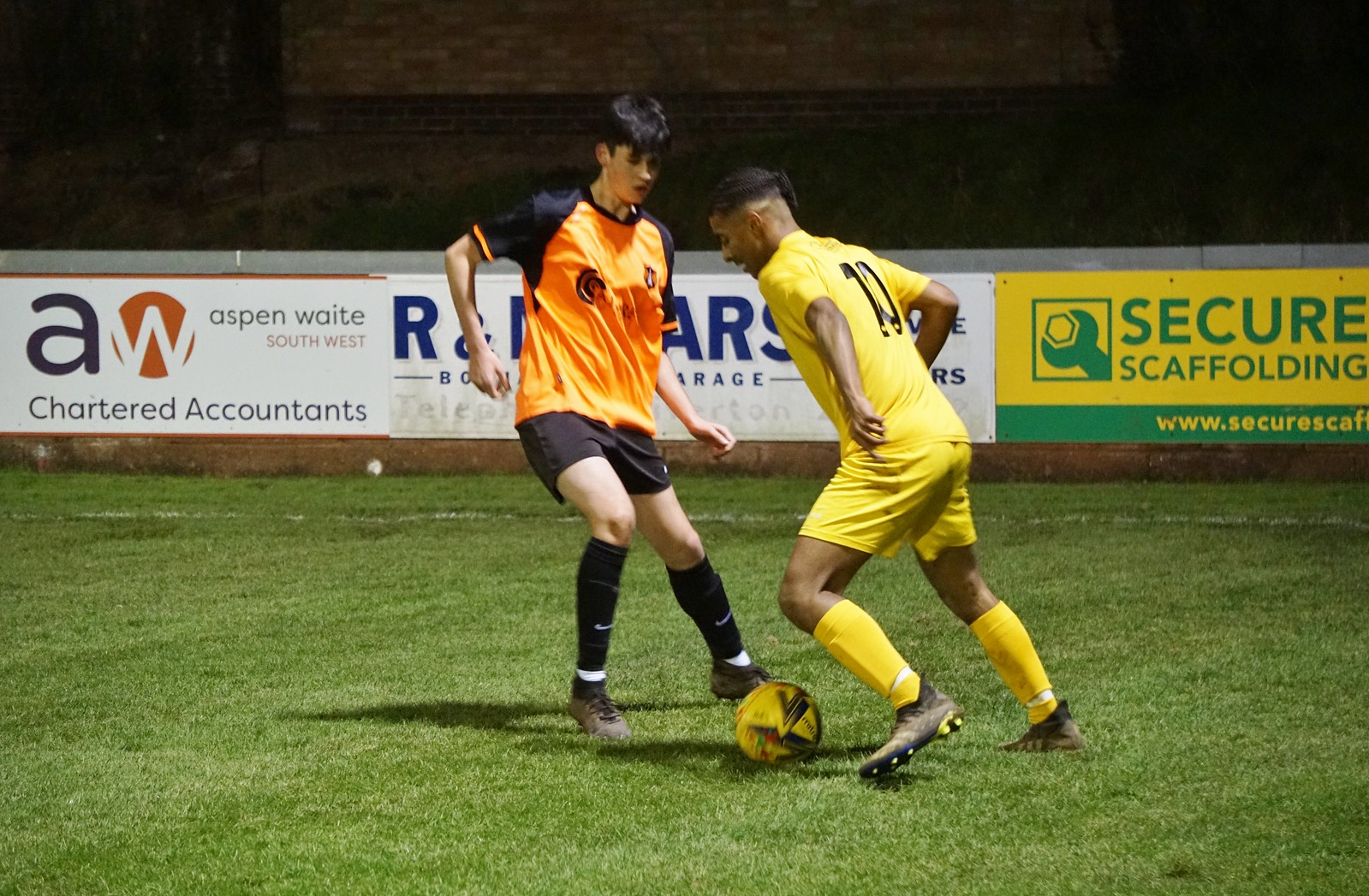In the nighttime image, two soccer players are captured on a green grass field with white lining marking the borders. A barrier wall surrounds the field, adorned with various advertisements like "A.W. Aspen Waite Southwest Chartered Accountants" and "Secure Scaffolding," among others. The player on the left, dressed in an orange jersey with black sleeves, black shorts, and black socks, has dark hair and is currently in possession of the yellow soccer ball with black accents. He is positioned lunging forward with bent knees and arms to the side. Opposing him, the player on the right is in a defensive stance, wearing a yellow jersey with a black number 10 on the back, yellow shorts, yellow socks, and black shoes, leaning back with bent knees. The scene is illuminated by the dark sky, highlighting the intense moment of competition between the two athletes.